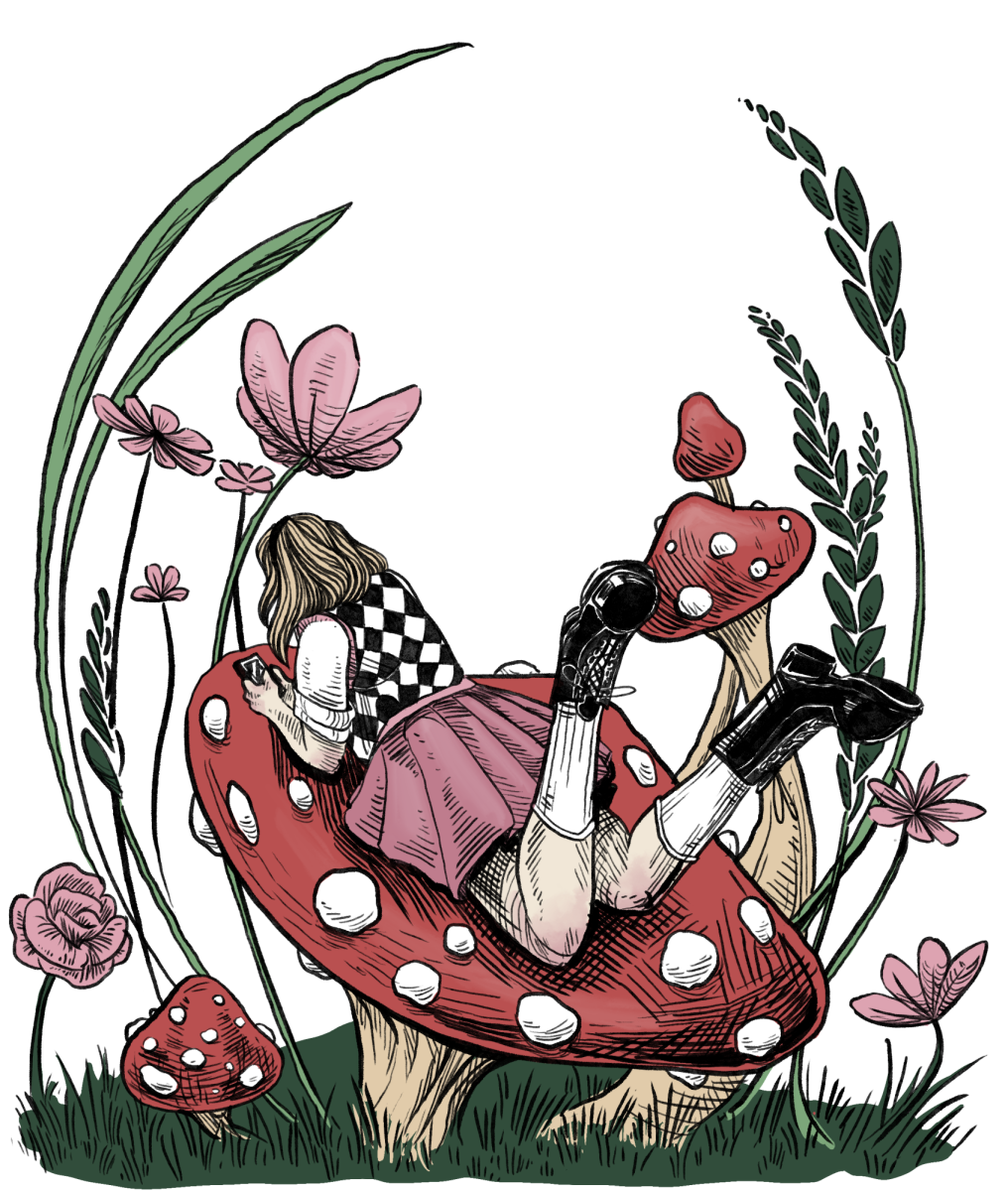The image is a detailed digital drawing that showcases a girl with blonde hair lying on her stomach atop a giant red mushroom, which is adorned with white spots. She is dressed in a checkered vest, a white short-sleeved shirt, a pink pleated skirt, and black ankle-length boots, and she is holding a cell phone in her hands, looking at it intently. The scene has a whimsical, Alice in Wonderland vibe, with a patch of green grass at the bottom and various other mushrooms of different sizes around her, their long tan or yellow stems reaching upward. To the left of the main mushroom, there is a smaller mushroom and a blooming rose, while to the right, tall dandelion-like flowers and additional mushrooms with extended stems add to the enchanting scene. The background is predominantly blank white, placing full emphasis on the colorful and imaginative elements centered around the girl and the mushrooms.